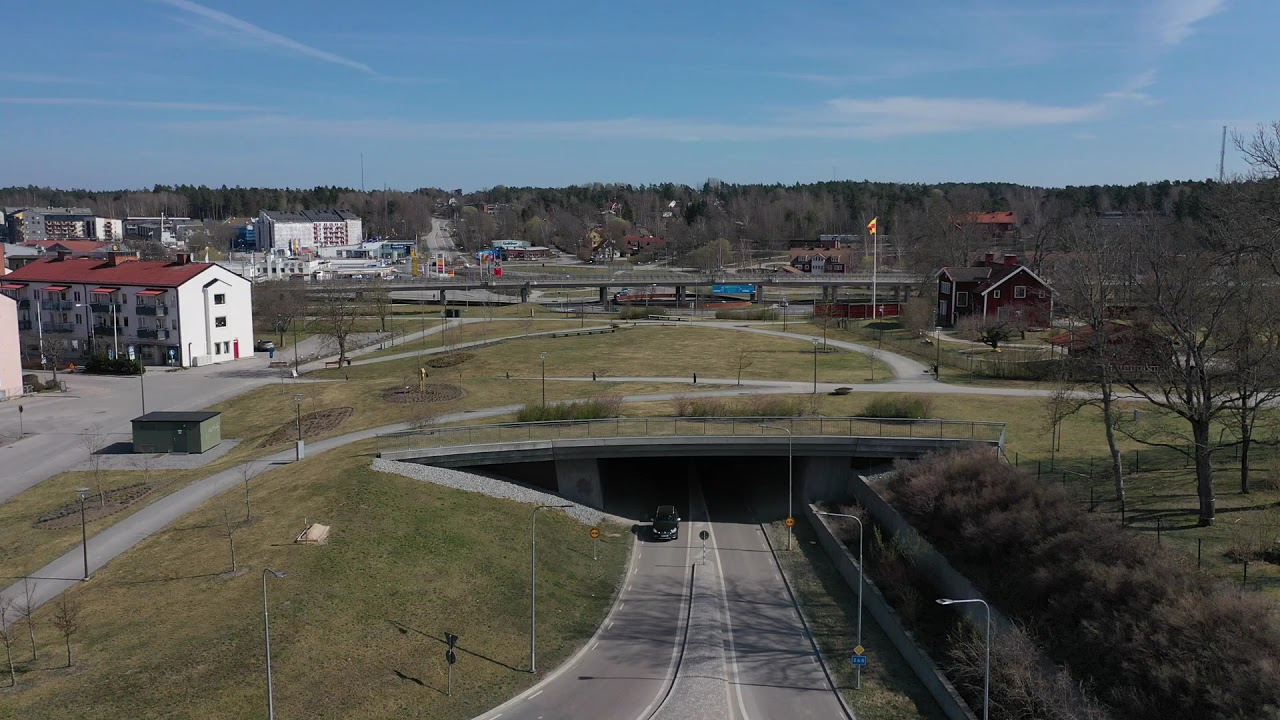A scenic aerial photograph captures a quaint rural town surrounded by green hills in the distance. The bottom of the image reveals a two-lane street, which intersects with an underpass forming a bridge that doubles as a pedestrian walkway with a small park area on top. Up close, streetlights and railings are visible along the road. 

To the left, there's a multi-storied building with a red roof that resembles a hotel, while on the right, a two-story structure with red walls and a grey roof looks like a church, despite lacking a cross. The middle of the photo features a black car emerging from the underpass on the right side of the road. 

Throughout the town, various three-story buildings can be seen, and off to the right center, a flagpole bearing a yellow flag with a red stripe stands prominently. The background is lined with mostly barren trees, suggesting a wintertime setting, and the sky above is lightly clouded but predominantly blue.